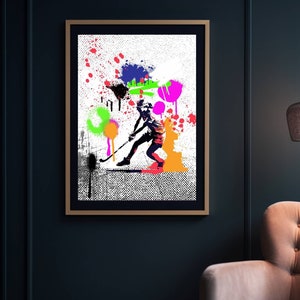A detailed photograph captures a vibrant painting hanging in a sophisticated living room with black-painted walls. In the lower right corner, a tan chair subtly enters the frame, adding an element of warmth to the setting. The painting, centrally positioned, is framed with a luxurious gold rim and a sleek black mat, emphasizing its bold presence. The artwork itself features a white background splattered with an array of dynamic colors, creating a sense of movement and energy. At the heart of the painting, a young woman, depicted in mid-action, is playing field hockey. Her figure, in motion with a stick in hand, appears to be running on a field marked with lines, surrounded by vibrant splashes and shapes of color that inject vitality into the scene.